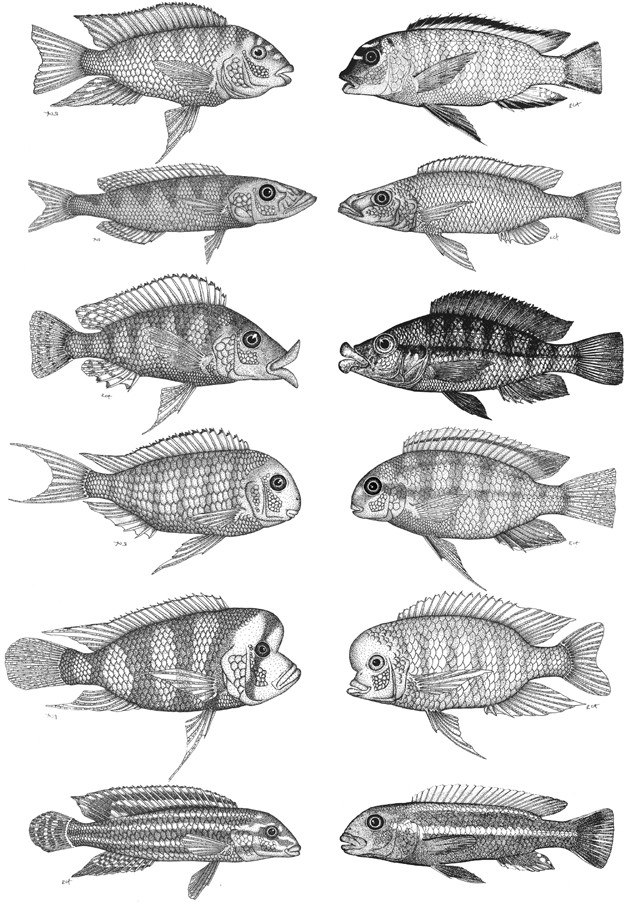This illustration features a composite of 12 meticulously detailed, black-and-white sketches of various fish species. Arranged in six rows, the fish on the left side face right, while those on the right side face left, creating a symmetrical design where the fish appear to confront each other. Each sketch showcases the unique characteristics of lake and river fish, with some displaying bulbous heads and others resembling small pike or other slender species. The assortment includes both thin and slightly plumper fish, influencing the visual balance of the composition. Notably, tiny, tidy writing is present next to most fish, except for two: one in the lower right and another in the third row from the top. The meticulous detail in the sketches suggests the use of reference photos, and the monochromatic palette adds to the lifelike quality of the artwork, set against a pristine white background.